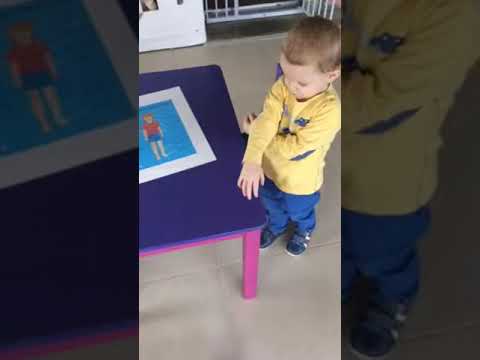In the living room setting, an image presents a triptych layout with blurred, enlarged elements on the left and right wings that serve as a grayish border. The main focus is on the centered, clear image of a toddler, dressed in a yellow long-sleeve shirt adorned with blue dinosaur designs, blue pants, and black sneakers, standing on a brown tile floor. The child has light brown hair and is positioned with his right hand on a small, child-sized table while his left arm is crossed underneath. The table, which has purple or pink legs and a dark blue or black top, holds a white-bordered drawing of a child wearing a red shirt and blue shorts against a blue background. In the background, a white door and a gate or grill are partially visible, emphasizing the interior setting of the room.